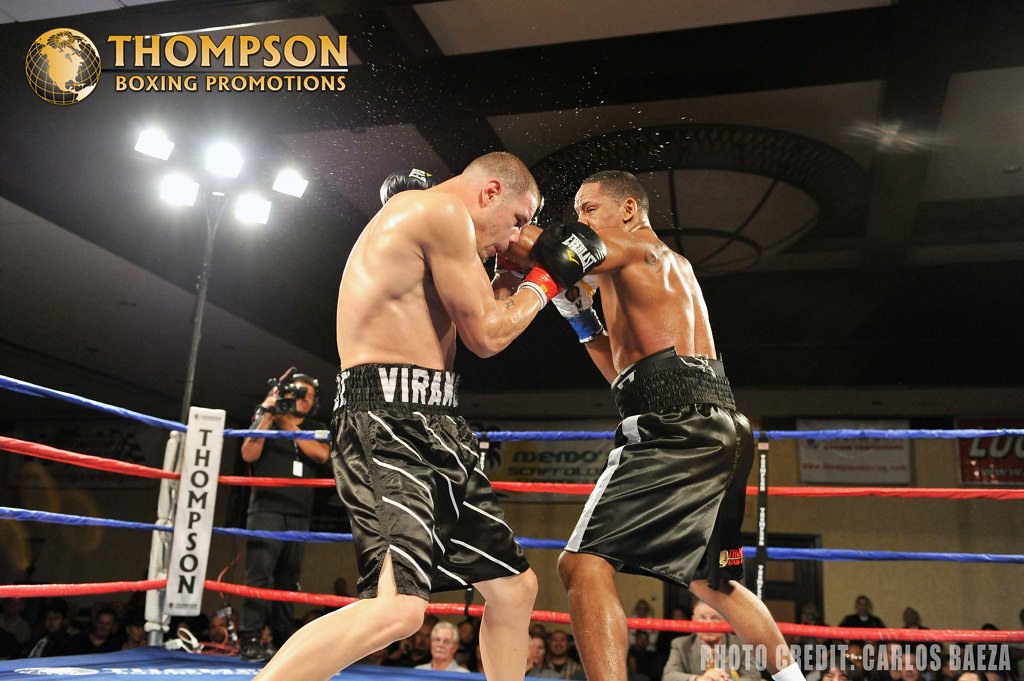In the photograph, two shirtless men are intensely boxing in a ring. Both are wearing large black boxing shorts, with the boxer on the right having a light gray stripe on his shorts and the boxer on the left featuring small gray diagonal stripes. The boxer on the right is in the midst of landing a punch on the left boxer's nose. Overhead, a bright stand with five spotlights illuminates the scene.

In the upper left corner of the image, a black and gold globe logo is prominently displayed, accompanied by the gold text "Thompson Boxing Promotions" just to its right. The boxing ring is bounded by ropes that alternate between blue and red from top to bottom. A white corner post stands at the ring side, adorned with the word "Thompson" in vertical black lettering. Positioned behind the ring, in the left background, a cameraman dressed in a dark shirt and pants captures the action with a camera on his right shoulder. In the bottom right corner of the image, an opaque white text notes "Photo Credit Carlos Beza."